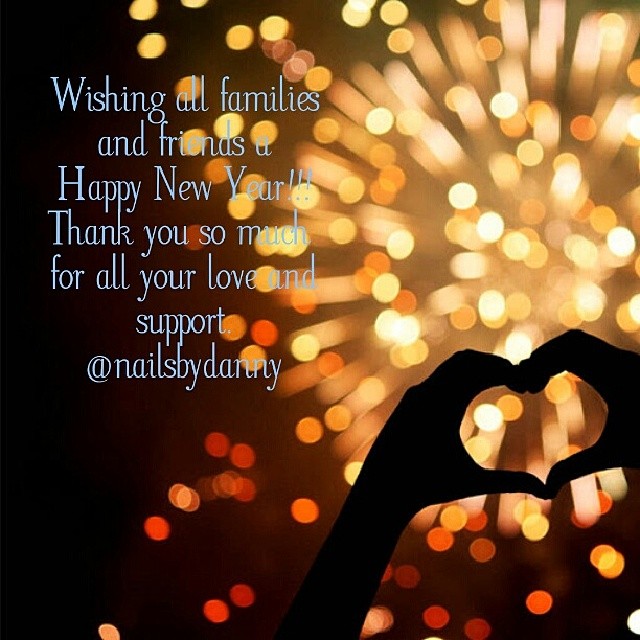The image depicts a promotional holiday celebration post, likely for a social media or website, from a store called "Nails by Dani." Against the backdrop of a night sky illuminated by yellow, orange, and gold fireworks, a person's hands form a heart shape in the foreground. The heart shape, created by connecting their thumbs and forefingers, is silhouetted against the vibrant firework display. To the left of the scene, in light blue text, the message reads: "Wishing all families and friends a Happy New Year. Thank you so much for all your love and support. At Nails by Dani." The background of the image transitions from black to brown as the fireworks light up the night. This festive image combines the warmth of personal sentiment with the visual delight of New Year's fireworks.